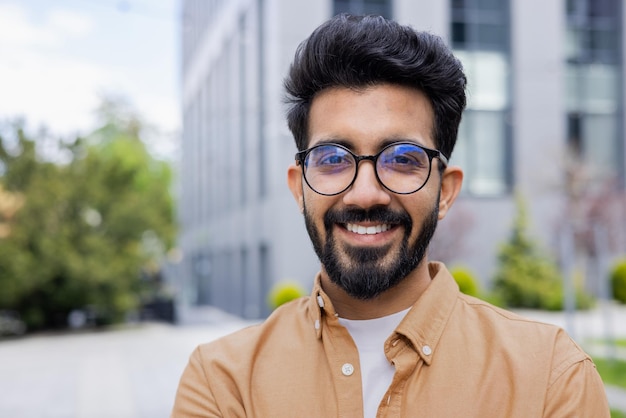In the background of the image, lush green trees stand tall alongside a modern silver office building with numerous windows, creating a scenic and professional atmosphere. The primary focus of the image is a young man, likely in his early 20s, who appears to be indoors, positioned with his back to a window. He has slightly tanned skin, a well-groomed dark brown to black beard and mustache, and black hair styled straight up, reaching several inches high. He is dressed in a white t-shirt beneath a light brown, almost orange-brown collared shirt adorned with buttons. The man is also wearing black-rimmed glasses, through which faint reflections of what seem to be one or two computer monitors are visible. This suggests that the photo may be his professional headshot, potentially featured on a company’s website.